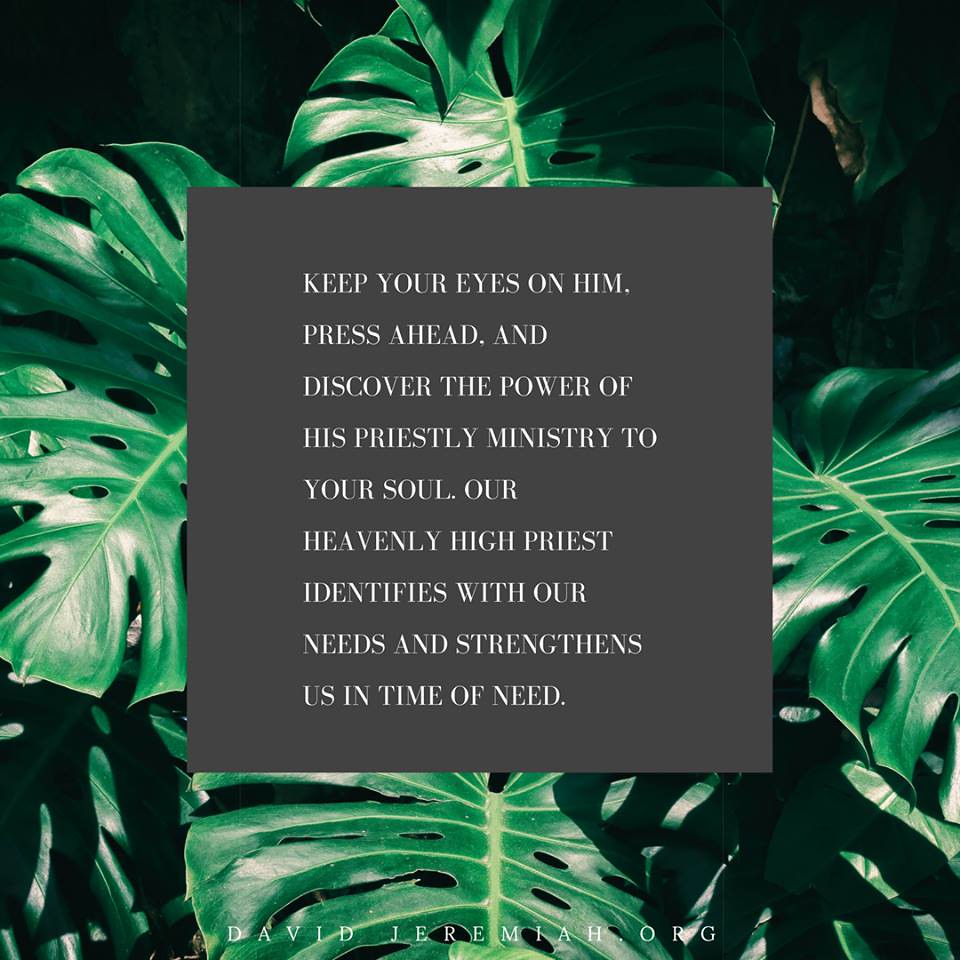The image features a background of large green fern leaves, filling the frame with leaves extending towards each edge: one leaf reaches upward, another to the left, one to the right, and one downward. These primary leaves are overlaid on a shadowy backdrop of darker, faded-out foliage. A prominent dark grey textbox occupies the center of the image, displaying an inspirational message in all caps white font. The text reads, "KEEP YOUR EYES ON HIM, PRESS AHEAD AND DISCOVER THE POWER OF HIS PRIESTLY MINISTRY TO YOUR SOUL. OUR HEAVENLY HIGH PRIEST IDENTIFIES WITH OUR NEEDS AND STRENGTHENS US IN TIME OF NEED." The text is formatted like lines of a poem but doesn’t rhyme. At the bottom of the image, the website "DAVIDJEREMIAH.ORG" appears in white uppercase font. The overall composition gives a sense of serene encouragement, tying spiritual strength to the natural imagery.